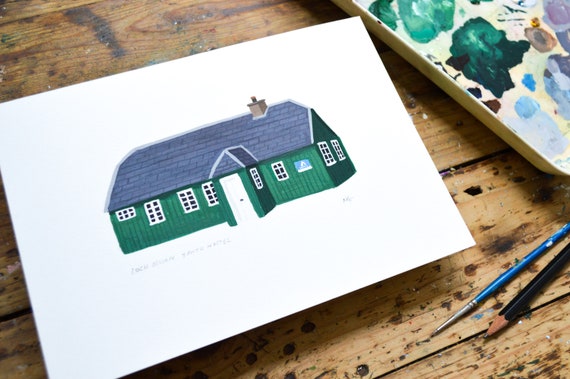This is a detailed photograph of an amateur drawing placed on a rustic wooden surface with various shades of brown. The focal point is a white piece of paper featuring a green farmhouse or barn-like structure. The building has a blue rooftop with a small brown chimney in the top right corner and is adorned with 7 windows framed in white and painted black. A white door juts out from the front. Surrounding the drawing are traces of paint and a painter's tray with an assortment of colors. In the bottom right corner of the image, there lie two paintbrushes, one blue and one black, along with a pencil. The drawing itself is tilted, with the right corner higher than the left. There is also some indistinct writing near the lower left and lower right sides of the paper, possibly the artist's signature or a print number. The entire setup is laid upon a wooden table, further emphasizing the art's rustic and homemade nature.